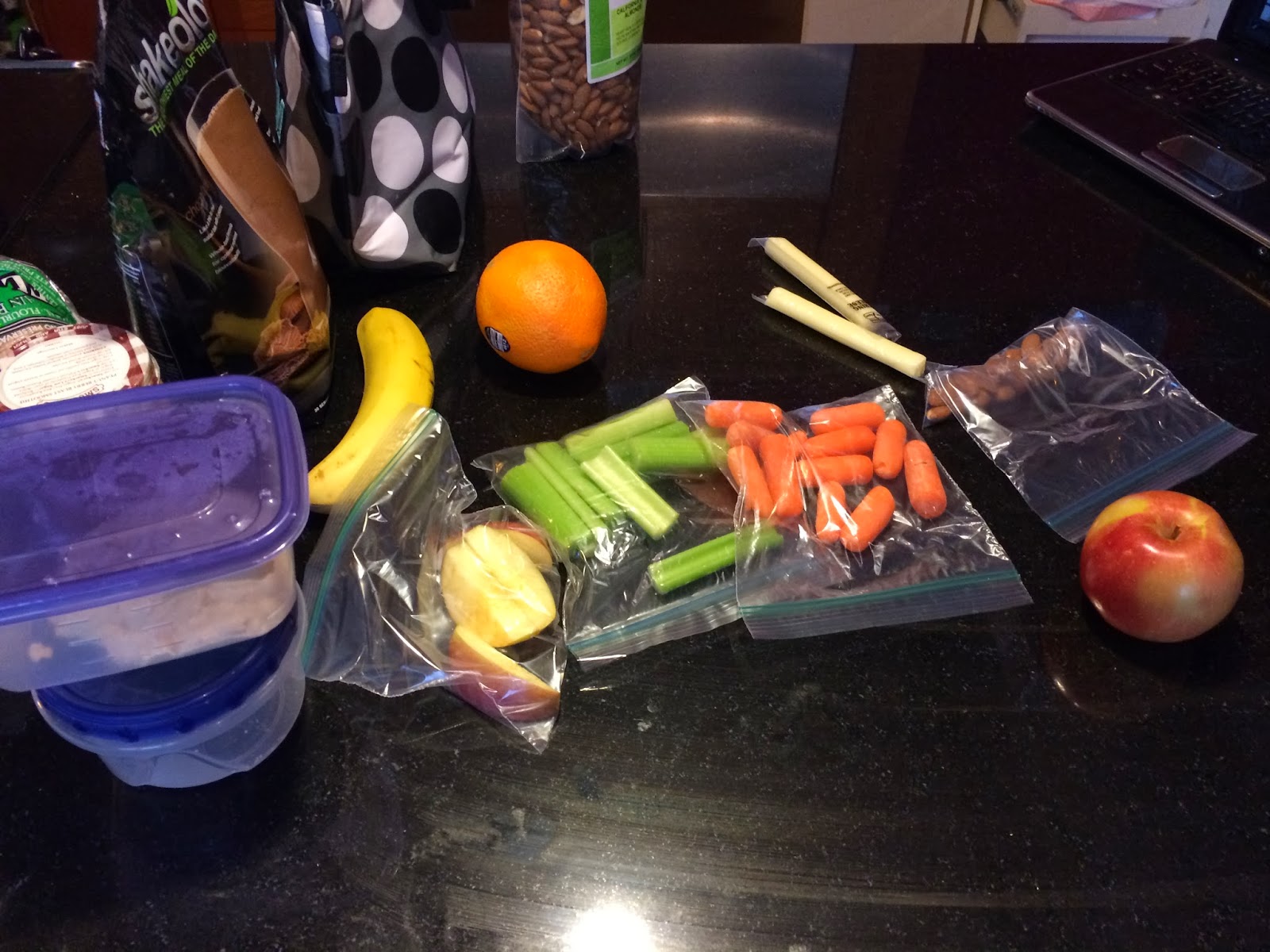In this image, a black table serves as the base for a variety of items neatly arranged. On the left side, there is a square, clear plastic container with a purple lid sitting on top of a round, clear plastic container with a blue lid. To the right of these containers, a red apple is placed next to a clear plastic bag that appears to contain some brown nuts. Adjacent to this bag is another clear plastic bag filled with carrots, followed by a bag of green celery, and then a bag containing chopped apples, revealing their yellow interior. Just above these, a yellow banana lies next to a vibrant orange. Positioned at the top of the display is a clear bag suspected to be filled with brown almonds. On the far left, a round white wrapper with red and white edges is visible. Finally, a polka-dot patterned item with black, white, and gray coloration appears in the background, along with what seems to be a brown arm wearing a black t-shirt with white lettering on it.